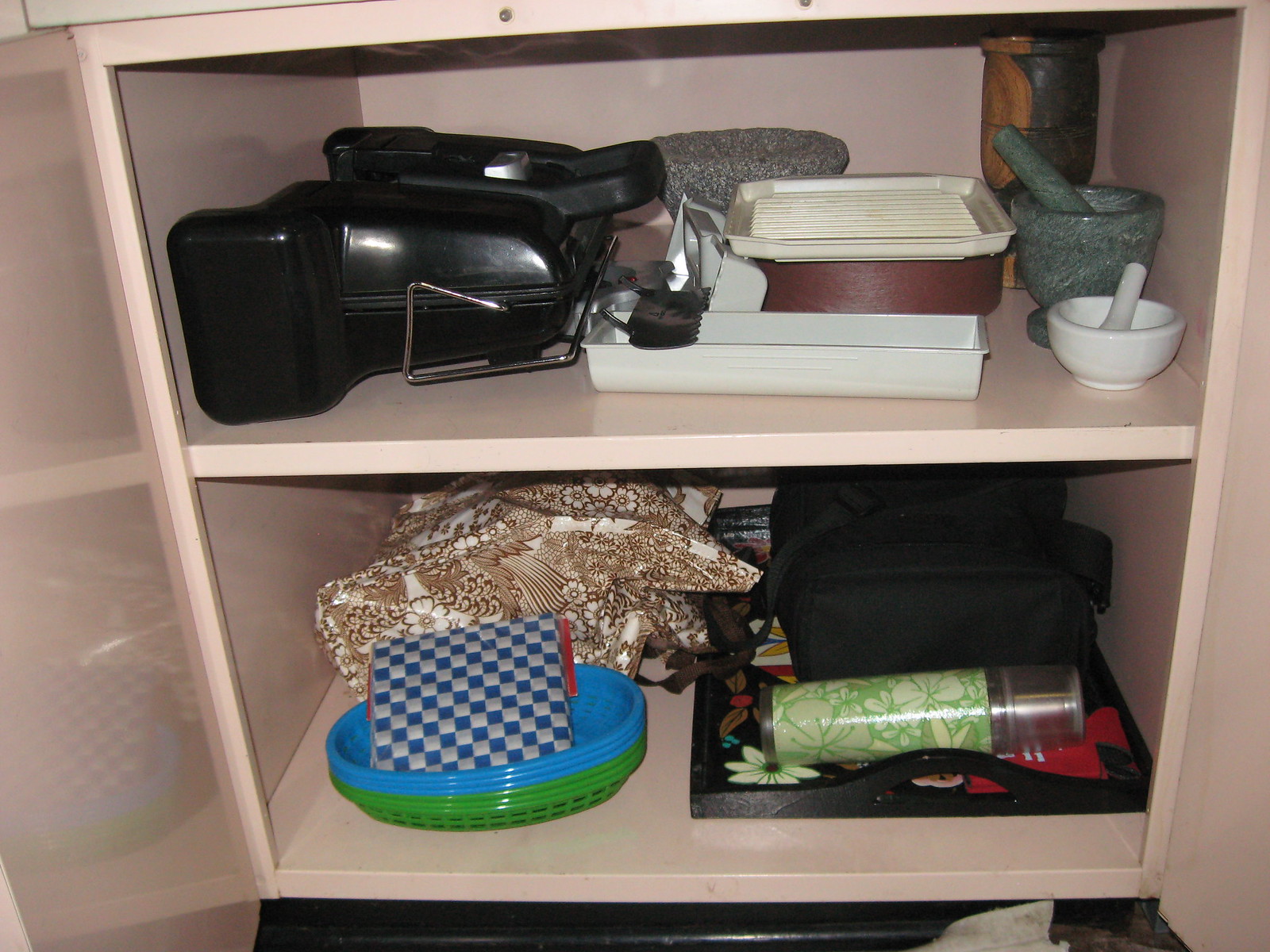Here is a cleaned-up version of the caption:

In the close-up photo of an open kitchen cabinet painted in a light pink hue, the interior and doors are all pink. On the upper shelf to the right, there are two mortars and pestles—one white and one gray. Next to them is a square container with a plastic lid, which could be used for holding sandwiches, although it appears slightly larger. A long rectangular white tray is also visible on this shelf. Beside these items, there's a large black appliance encased in a cover, its exact function unclear.

On the lower shelf, there are plastic baskets resembling plate liners. Additionally, a set of blue and white checked napkins is present, with a brown and white folded cloth behind them. A black, possibly insulated, lunch bag sits next to a green and ivory thermos, which appears to have a silver cap. Lastly, there's a black tray with a floral insert.